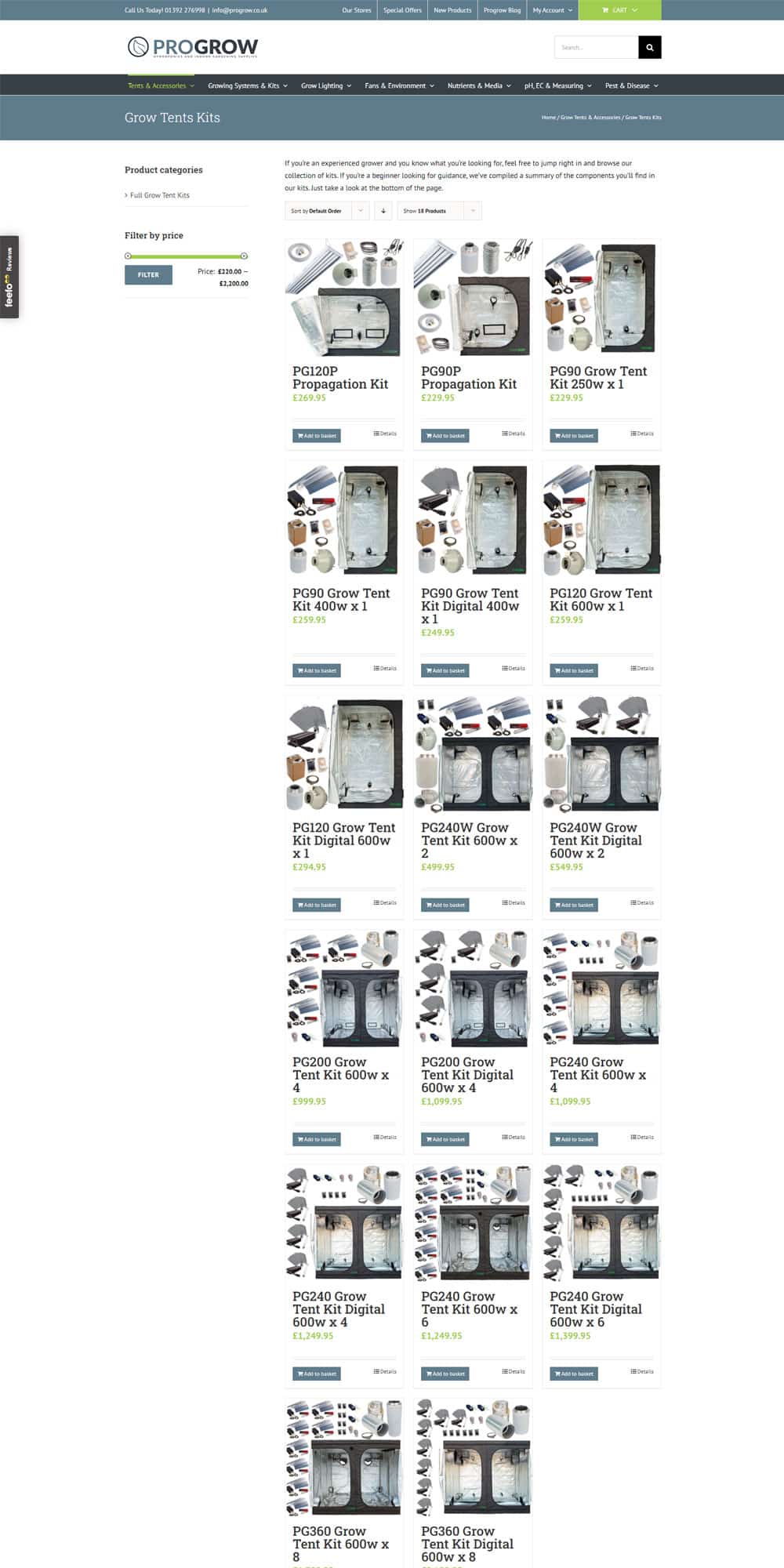The webpage displayed belongs to ProGrow, identifiable by its logo situated in the upper left-hand corner. The logo features the word "PROGROW" in all capital letters, with "PRO" rendered in a lighter blue and "GROW" in a darker blue, set against a white background. Adjacent to the logo is another logo element. The top of the page hosts a slim blue bar with text that is too small to decipher. Below the ProGrow logo, a dark bluish-gray navigation bar likely contains pull-down menus, although the minuscule text makes their labels unreadable. The currently active tab appears to focus on "Grow Kits."

Directly underneath this tab, there's a series of clickable links, including one labeled "Filter." This filter presumably allows users to narrow down their search results. The page displays a total of 17 results, organized in six rows with three items per row, except for the final row, which contains only two items.